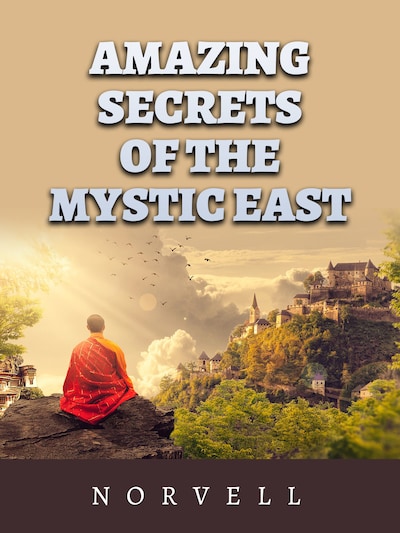The image is a detailed book cover with a light terracotta brown background and the title "Amazing Secrets of the Mystic East" prominently displayed in bold white serif font at the top. The cover features an evocative scene with a monk dressed in an orange cloak sitting with his back turned to the viewer. He is perched on a rock that overhangs a lush green forest, with his gaze directed towards a sky filled with fluffy white clouds and several black birds mid-flight. Sunlight streams through the clouds from the left side of the image, illuminating the serene setting. To the right of the monk, a castle-like structure is visible amidst the trees, situated on a hill dotted with older buildings that extend up the mountainside. The scene offers a majestic view overlooking the towering heights and rolling clouds. At the bottom of the cover, the name "Norvell" is displayed in white lettering atop a dark brown stripe.